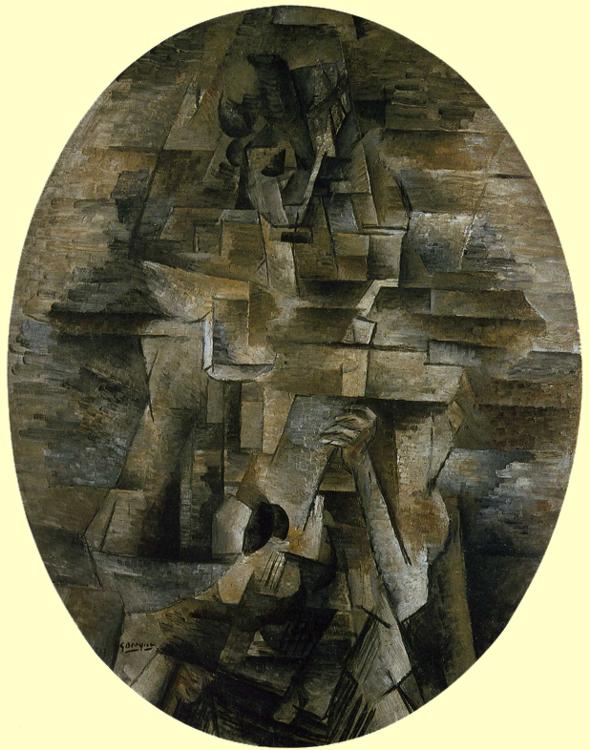The image depicts an abstract oval-shaped sculpture with a hand extending from it, seemingly grasping or interacting with a blocky, three-dimensional structure. The sculpture is a composition of stacked blocks and intricate shapes, primarily in shades of gray, blue, and brown, with hints of green and black. The hand appears to emerge from the lower right side of the image, resembling claws trying to grasp a rectangular object with a hole at the bottom. Above this, a ram’s head or a similar form protrudes from the structure. The oval is bordered by a pale, off-white or peach color with a subtle yellow tint, reminiscent of light banana. In the bottom left corner, there are small initials or a name, indicating the artwork's creator. The overall scene is set against a yellow border, adding a striking contrast to the intricate central composition.